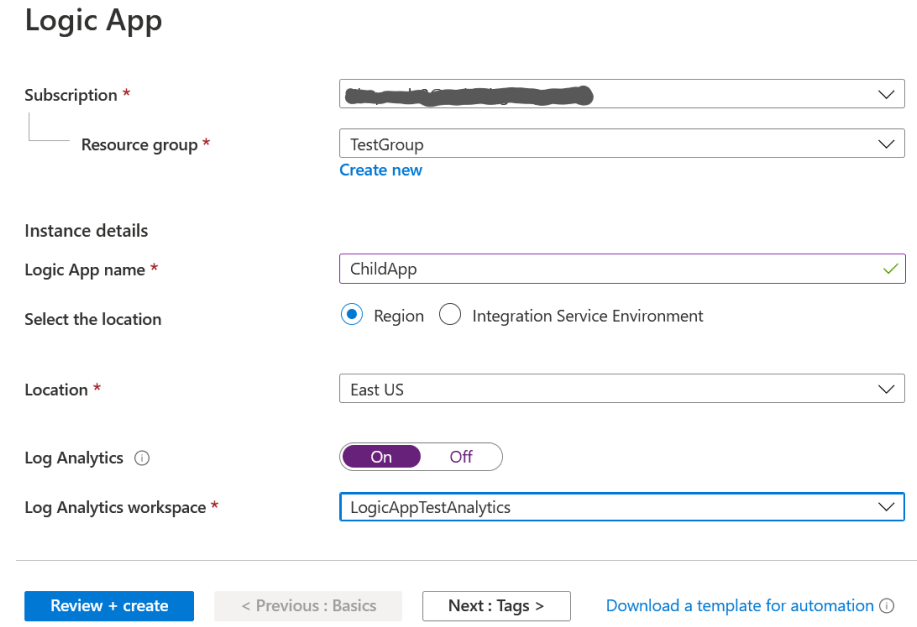The image showcases a detailed form interface for configuring a Logic App. 

At the very top left corner, "Logic App" is prominently displayed in bold black font. Below, the interface lists several required fields indicated by a red asterisk: "Subscription," "Resource Group," "Instance Details," "Logic App Name," "Location," "Log Analytics," and "Log Analytics Workspace." 

Further down, a blue button labeled "Review + Create" is present. 

In the middle section, the form includes a white rectangle with blacked-out text, followed by a rectangle with "Test Group" in black letters. Below it, "Create New" appears in blue text, and another rectangle labeled "Child App" is shown.

Further details include options for "Region" and "Integration Service Environment," each prefixed by a circle. The "Region" circle is highlighted with a blue outline and a filled blue circle. A rectangle beneath this displays "East USA."

To the right, there's a toggle switch for an On/Off option, outlined in gray; the "On" position is marked in purple, while "Off" is displayed in black text.

Towards the bottom, a blue rectangle reads "Logic App Test Analytics," followed by buttons labeled "Next" and "Tags." Adjacent to them, a blue link allows users to "Download a Template for Automation."